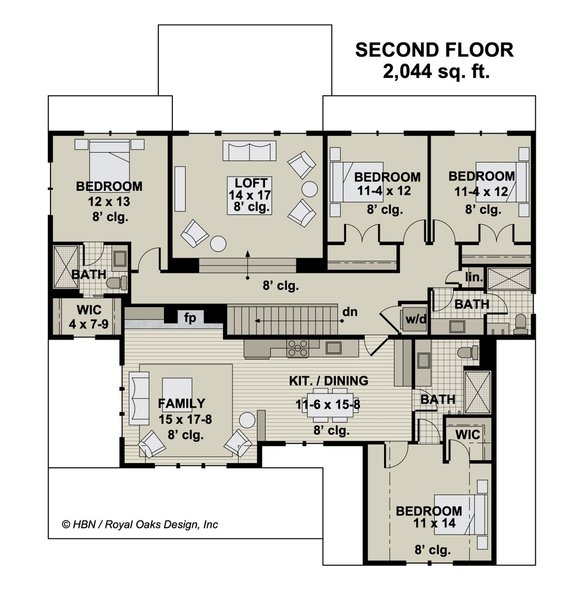This detailed architectural drawing illustrates the second-floor plan of a home, encompassing an area of 2,044 square feet. Highlighted in black letters at the top of the illustration is the label "Second Floor, 2,044 SQ FT." The layout includes a series of clearly labeled rooms and dimensions: a family room measuring 15 by 17 feet, adjacent to a kitchen and dining area of 11.6 by 15.8 feet. Flanking the kitchen on the right-hand side is a bathroom. 

Additionally, the floor plan features multiple bedrooms: one at 12 by 13 feet, another at 11 by 14 feet, and two identical bedrooms each at 11.4 by 12 feet. The loft space measures 14 by 17 feet, and there is a bath on the left-hand side near a walk-in closet (WIC) sized 4 by 7 feet. The bottom left-hand corner of the plan bears the copyright of HBN/Royal Oaks Design, Inc. 

The blueprint's background is white with elements rendered in shades of gray, brown, and black, providing a clear, concise representation of the home's second floor.